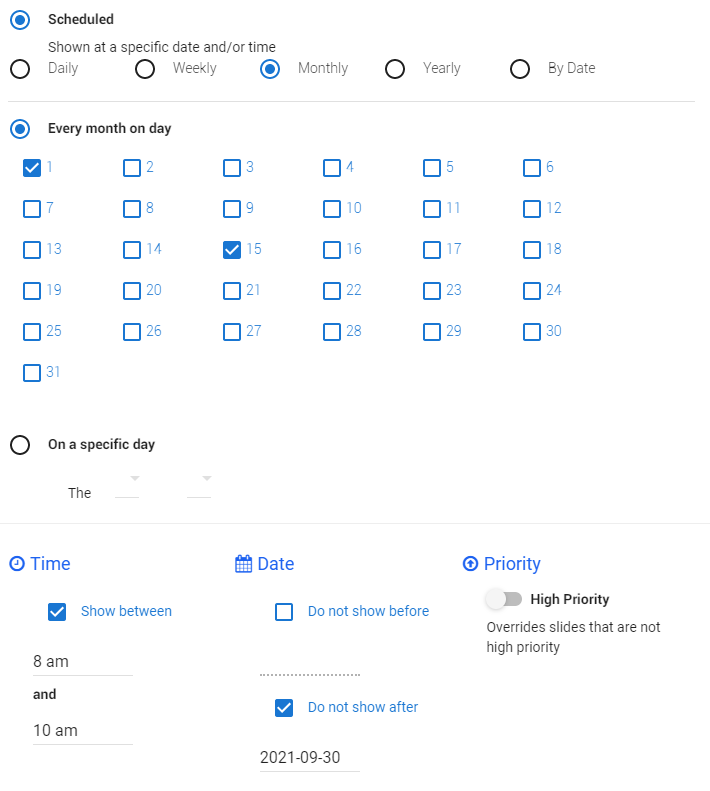This detailed screenshot of a calendar scheduling interface features a clean, white background. In the top left corner, a distinct white circle is outlined in blue, containing a blue dot in its center. Adjacent to this symbol, bold black text states "Scheduled." Below this heading, thinner black text reads, "shown at a specific date and/or time."

Continuing downward, five consecutive icons—circles with corresponding labels—represent various scheduling frequencies: "Daily," "Weekly," "Monthly," "Yearly," and "By Date." A thin gray line separates these elements from the section below.

Under this divider, a similar white circle with a blue outline and center dot reappears on the top left. Next to it, in black text, is the phrase "Every month on day." Below this, a grid displays numbers from 1 to 31, each with a checkbox to their left. Both the boxes for the 1st and the 15th are ticked. 

Following this, a black-outlined circle precedes text that reads "On a specific day." Directly beneath, the text "The" is followed by two drop-down menus for additional specificity.

At the bottom of the screenshot, blue text indicates further options: "Time," "Date," and "Priority." Additionally, more detailed scheduling settings are visible: "Show between," "Do not show before," and "High priority."